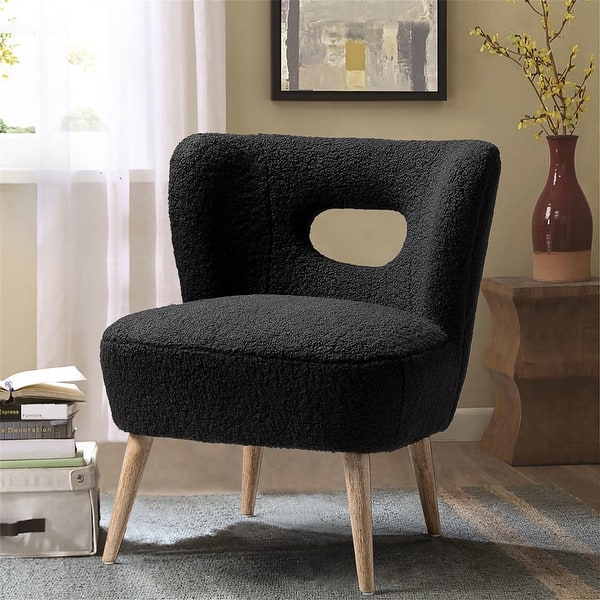A large, detailed photograph captures an intimate corner of a cozy living room. Dominating the center is a short, cushioned chair with four small light-wood legs. The chair’s plush seat and backrest are upholstered in black fabric, with an oval cutout in the center of the backrest giving it a distinctive look. It sits atop a gray area rug adorned with tan stripes, horizontally oriented on a light wood floor. 

To the right of the chair, there is a unique stone stand holding a ceramic vase—tan on the bottom and brown on top—sprouting long branches with light green leaves, possibly resembling pussy willows. A stack of reading materials, including books, rests on or near canvas storage boxes beside the chair. 

Behind the chair, the wall is painted a warm tan color and features an abstract painting in shades of gray, gold, and white, set in a narrow black frame. Adding to the serene ambiance, lacy curtains hang in front of a window on the upper left side of the image, with sunlight streaming through and illuminating a few visible branches outside.